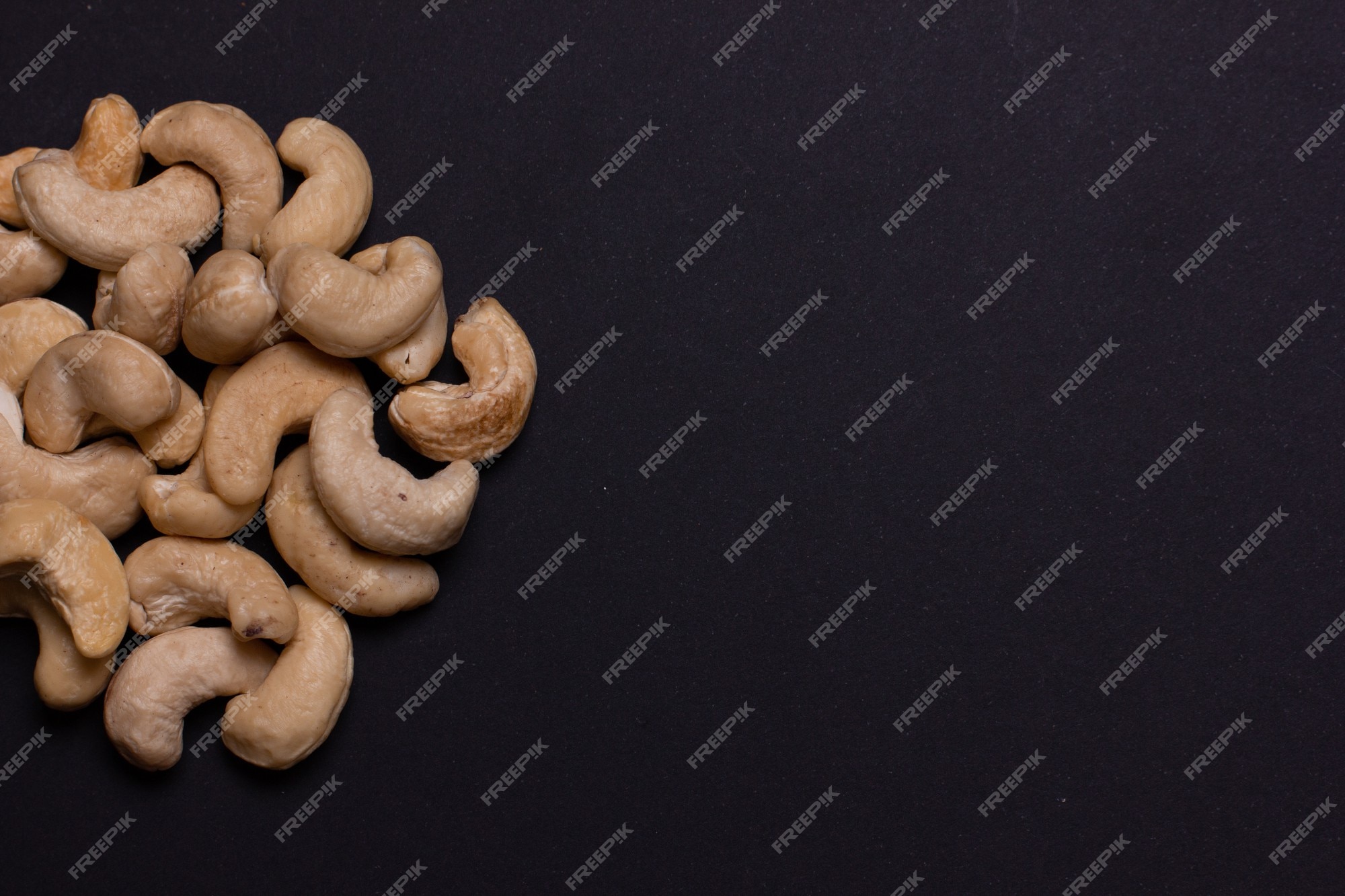This stock photo showcases roughly 20 shelled cashew nuts, tannish-light brown in color, stacked in a small pile towards the left side of a flat black background. The textureless backdrop accentuates the nuts, which appear plain without any salt or roasting. Diagonally spanning the image from the bottom left to the top right, a repeated watermark stating "freepik" in small white text covers the entire photo, serving as a prominent copyright indication tool.